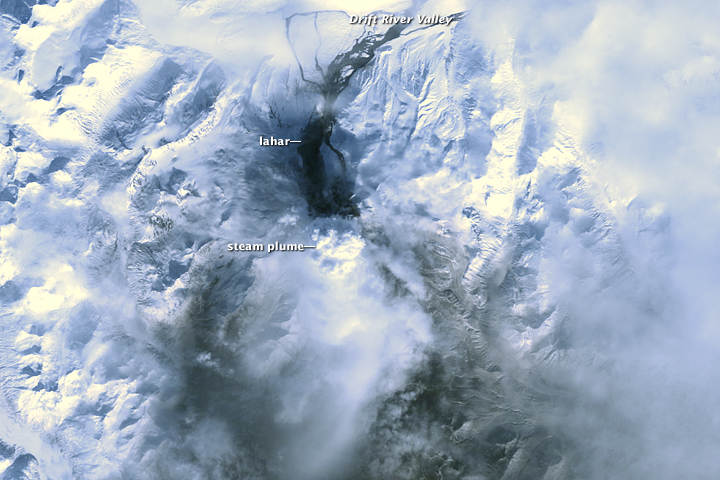An aerial, possibly satellite, photograph showcases a vast expanse of snow-covered mountain ranges in shades of white, light blue, gray, and brown. The right side and lower edge of the image feature partial cloud cover, adding to the dramatic, icy landscape. Dominating the upper half of the image is the Drift River Valley, centrally located with a distinctive dark streak, likely a river or water feature. This valley is marked by white text as "Drift River Valley" at the top, "Iyihar" approximately two-thirds down, and "Steam Plume" near the bottom, where a visible steam plume adds texture and intrigue. The image portrays photorealistic details, capturing the stark contrast of snow and possible volcanic ash, suggesting either volcanic activity or a deeply snowy region marked by natural elements.